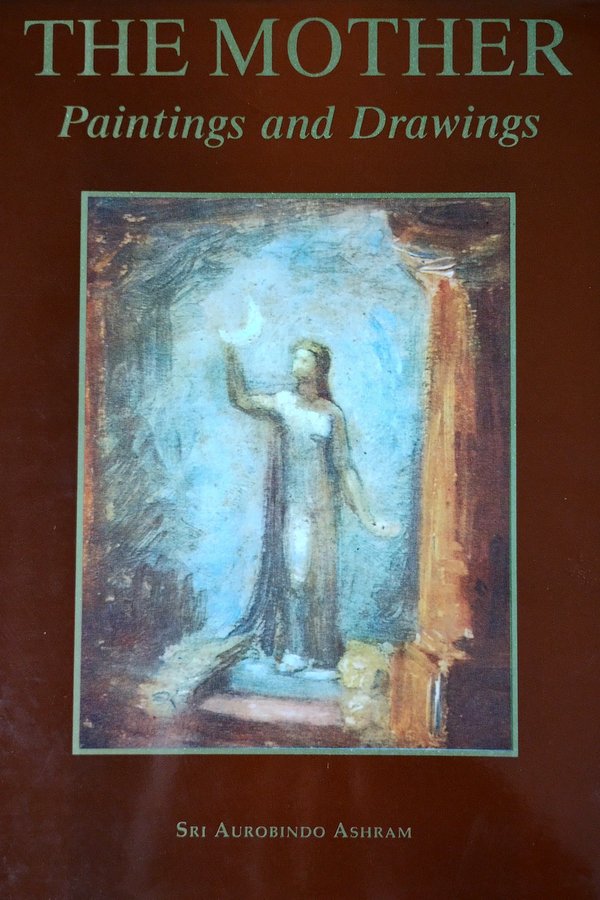The book cover titled "The Mother: Paintings and Drawings" by Sri Aurobindo Ashram features a deep brownish-maroon background. The title is prominently displayed at the top in a type font, colored in a blueish hue. In the center of the cover is a large, abstract painting bordered in teal to match the title and the author's name. The painting itself depicts a woman with dark hair, clad in a tan coat and white dress, standing majestically between two pillars. She has one arm upstretched toward a crescent moon, with the other arm slightly extended by her side. The background of the painting, crafted with choppy brush strokes, is a light blue, creating a dreamlike, almost stage-like setting beneath a moonlit sky. The author's name is centered at the bottom in matching teal.